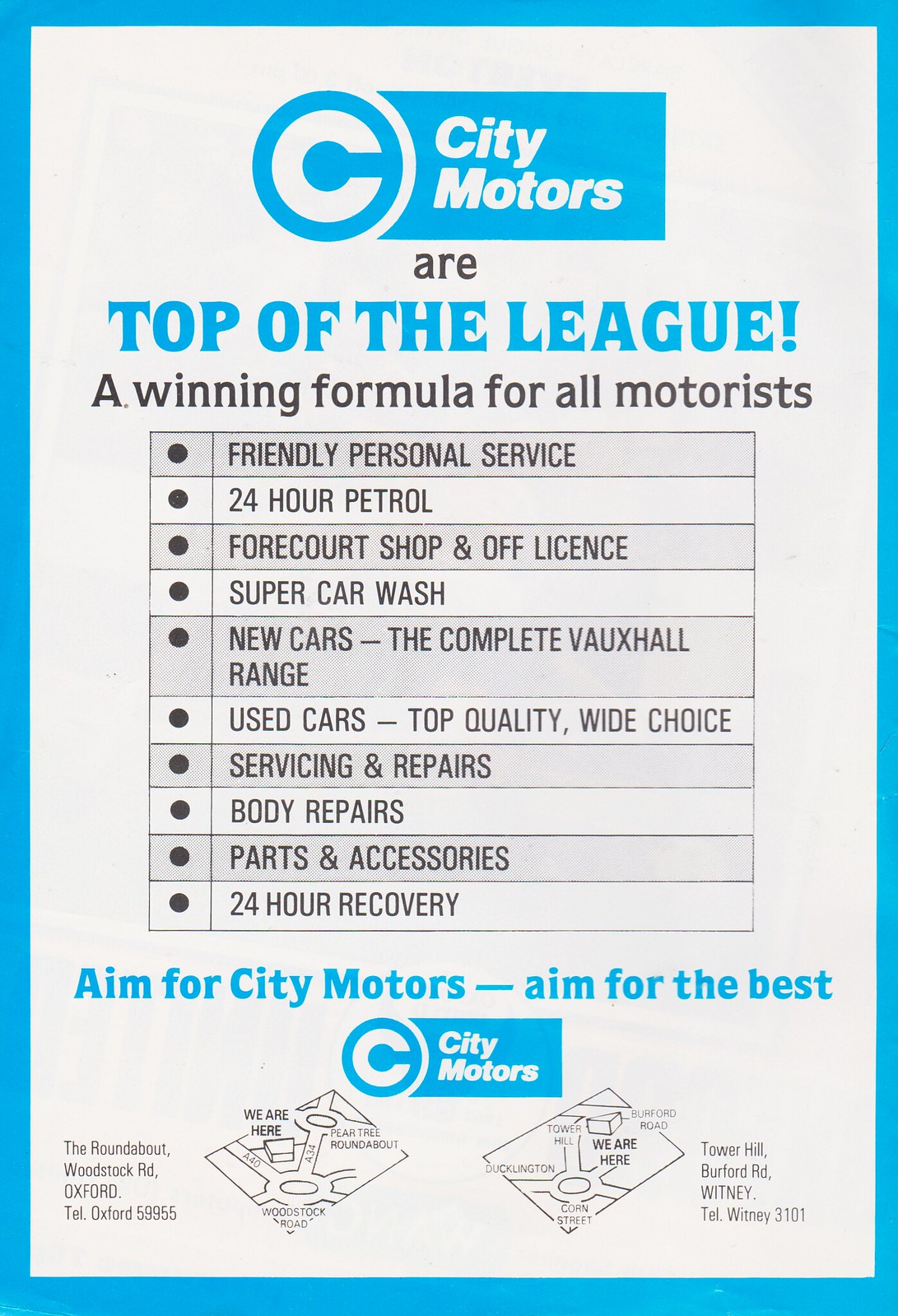This vintage-style advertisement for City Motors is a black-and-white printed page accented with spot color. The page is framed by a vibrant blue border, accentuating the brand's identity. At the top center, "City Motors" is prominently displayed in white font against a blue background, accompanied by a blue circle on the left featuring a white "C." Below, in an eyecatching blue font, the slogan "Top of the League!" stands out, followed by the claim in black: "A Winning Formula for All Motorists."

The ad boasts an array of services in a bullet-pointed table, including:

- Friendly Personal Service
- 24-Hour Petrol
- Four-court Shop and Off License
- Super Car Wash
- New Cars (the complete Vauxhall range)
- Used Cars (top quality, wide choice)
- Servicing and Repairs
- Body Repairs
- Parts and Accessories
- 24-Hour Recovery

At the bottom, the motivational line "Aim for City Motors - Aim for the Best" is printed in blue, alongside a repeat of the brand logo. Two intricately designed, slightly three-dimensional maps indicate the dealership locations at the roundabout on Woodstock Road, Oxford, and Tower Hill on Burford Road, Whitney, also providing respective contact numbers. This detailed composition of the ad ensures City Motors' dedication to premium service and accessibility is clearly conveyed.